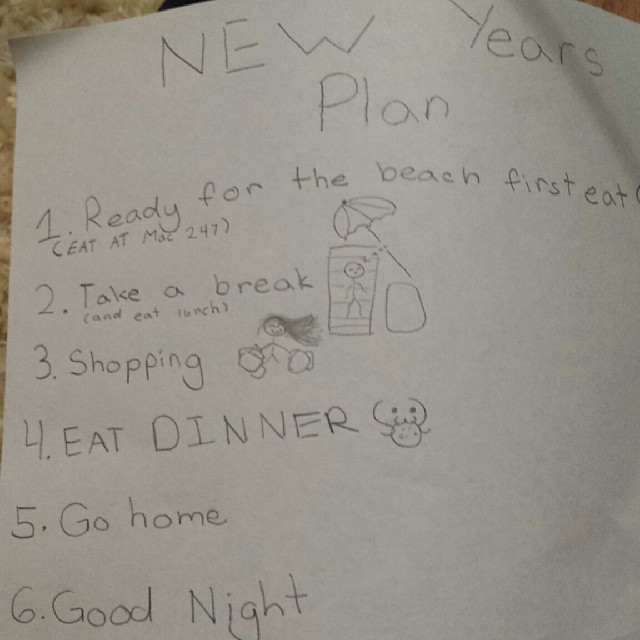The image displays a handwritten note on a white piece of paper laid against a tan, marble-like surface. The top of the note is headed with "New Year's Plan," followed by a list of six planned activities. 

1. "Ready for the beach" with "first eat (eat at Mac 24-7)" written underneath. 
2. "Take a break (and eat lunch)," accompanied by a doodle of a stick figure relaxing under a beach umbrella on a towel. 
3. "Shopping," illustrated by a stick figure with long hair carrying shopping bags. 
4. "Eat dinner," depicted with a doodle of a face eating what appears to be a cookie.
5. "Go home."
6. "Good night."

The mix of handwriting and simple illustrations adds a personal and whimsical touch to the detailed itinerary for New Year's Day.